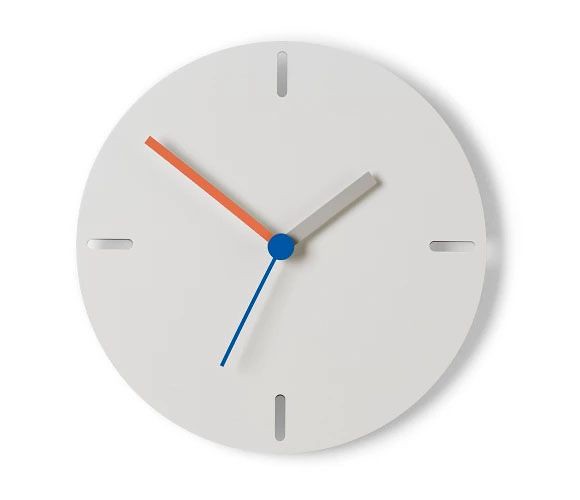This image features a very contemporary clock with a minimalist design. The clock face is white and lacks traditional numbers, instead featuring sleek silver lines at the 12, 3, 6, and 9 o'clock positions. The clock is designed with a raw edge, giving it a clean and modern look free of any rim. The clock hands are color-coded: the hour hand is silver, the minute hand is orange, and the second hand is blue. A blue dot marks the center where the hands connect, extending onto the second hand, adding a subtle touch of color. The overall aesthetic is reminiscent of a sand dollar, bringing a delicate yet sophisticated feel to its contemporary design.